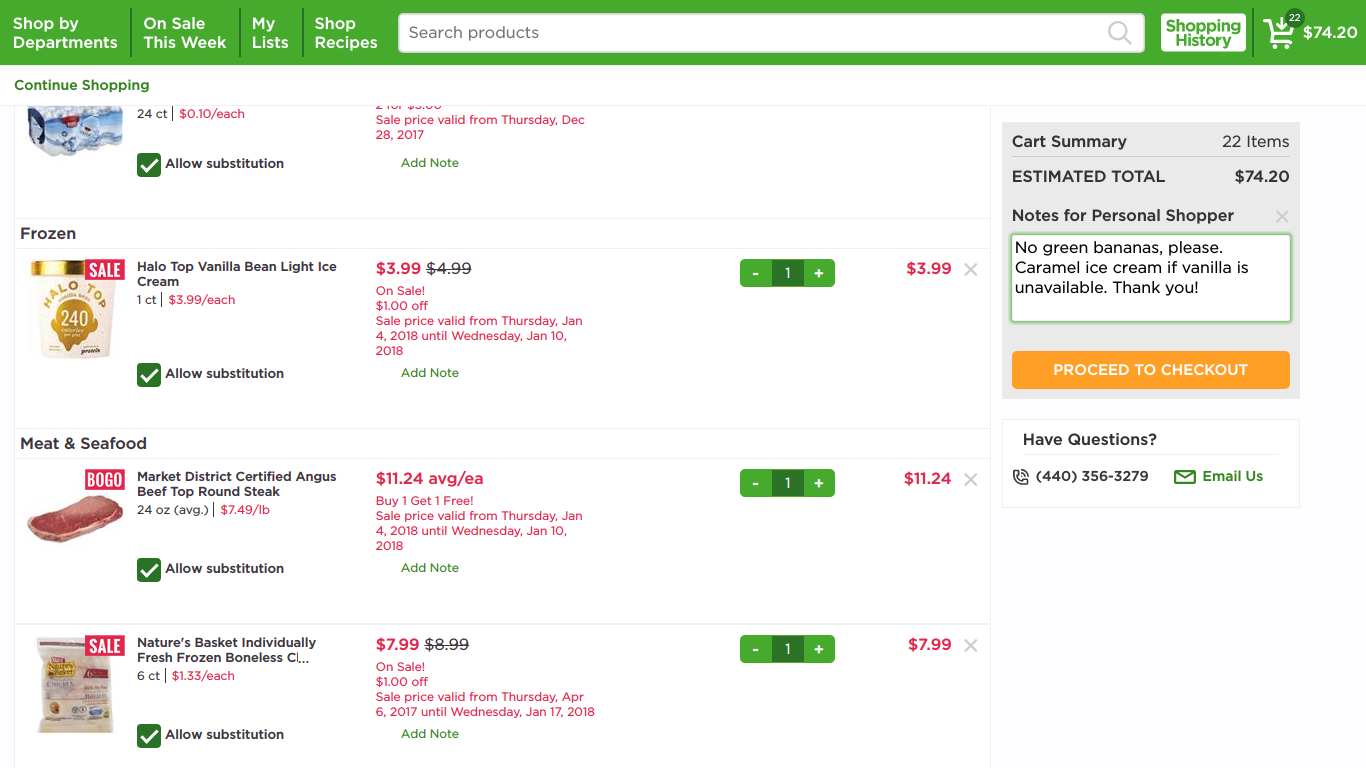The image displays a screenshot of a grocery shopping app on a computer, similar to Instacart. The app interface features a green navigation bar at the top, offering various categories such as "Departments," "On Sale," "Your Lists," "Shop Recipes," and "Shopping History." On the far right side of the bar, there is an icon indicating that there are approximately 20 items in the cart, with a current total of $74.20.

The visible items in the cart include sodas, ice cream, top round steak, and boneless chicken. Beneath the green navigation bar, a gray section appears on the right side of the screen, allowing shoppers to leave notes for their personal shopper. The notes listed include specific instructions: "No green bananas, please," "Caramel ice cream if vanilla is unavailable," and a polite "Thank you."